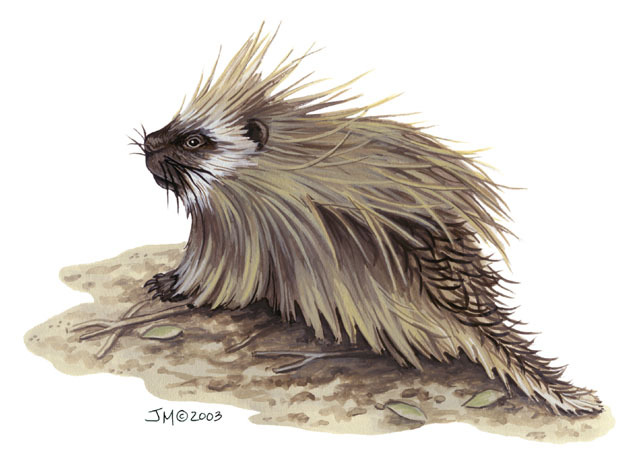This slightly diagonal painting from 2003, signed with the initials "JM" and a copyright symbol, depicts a side view of a porcupine against a white background that blends seamlessly into the white background of the task description. This brown and white porcupine, potentially appearing slightly wet, is positioned in a naturalistic setting featuring turf, ground, sticks, and a green leaf in the lower left corner. Its face, a darker charcoal gray with streaks of white, turns upward and to the left, while its long fur-like quills blend from black into white and tan. Two greenish-tan leaves are situated near the porcupine's tail on the right side. The tail itself is darker brown with short, fat quills lined in black and tipped with a slight white border. The initials "JM," encircled "C," and the date 2003 are inscribed at the bottom left in black, indicating the artist's signature.